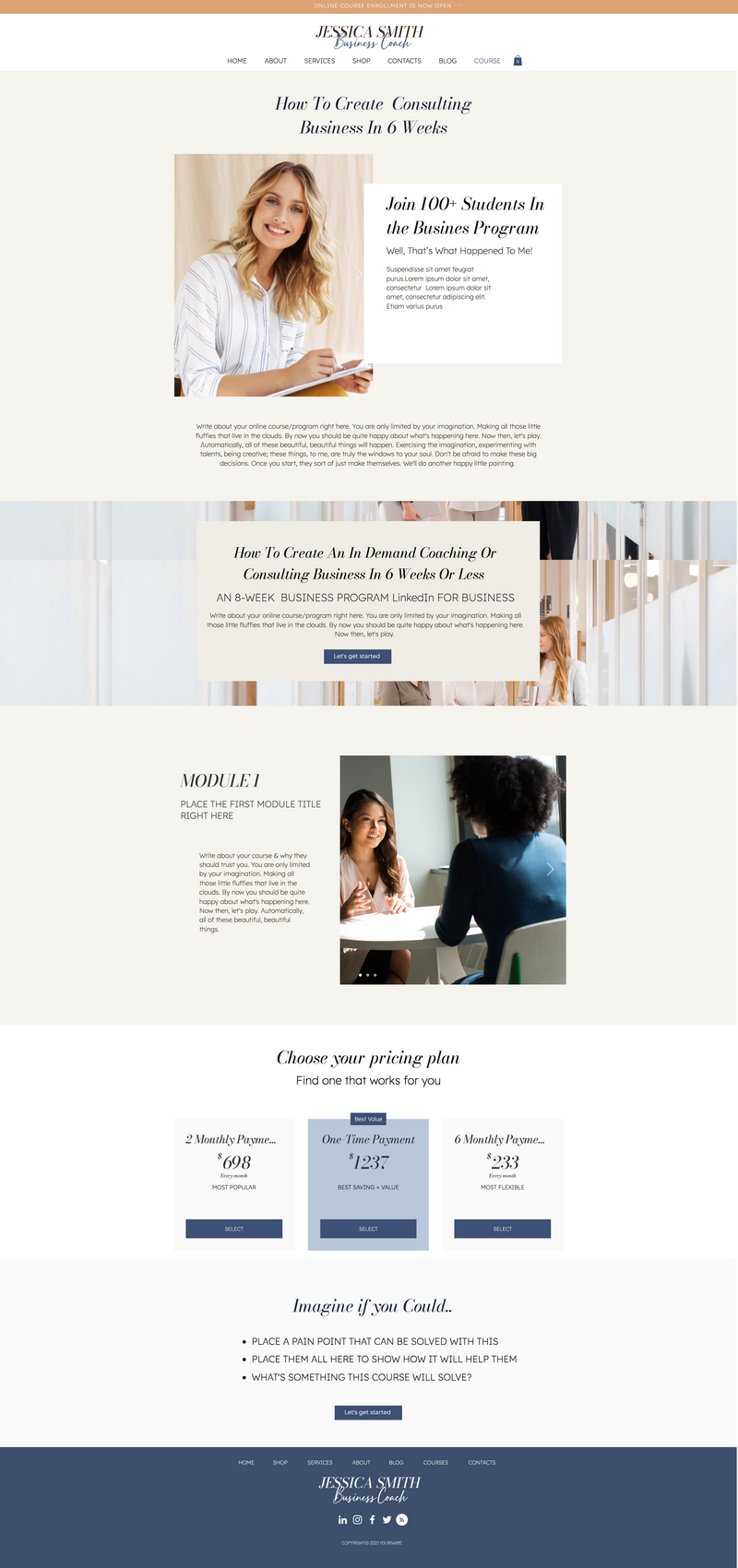At the very top center of the website, "JESSICA SMITH" is prominently displayed in an italic black font, all capitalized. Beneath this, the title "Business Coach" is written in a stylish blue cursive font. An orange banner stretches across the top from left to right, featuring the announcement "Online Course Enrollment is now open" in its center. 

Below the banner, there are seven navigation tabs: Home, About, Services, Shop, Contacts, Blog, and Course, listed from left to right.

Further down, on a slightly off-white cream-colored background, a large rectangular section is situated with the heading "How to Create a Consulting Business in Six Weeks" at the top center. 

Under this heading, there is an image of a woman with fair skin and ombre blonde hair, wearing a white shirt with vertical blue stripes.

To the right of the image, a box highlights the invitation, "Join 100+ students in the business program." Below this, in smaller font, it reads, "Well, that's what happened to me." Further down, placeholder text in another language or Lorem Ipsum is displayed: "Subsidies, Seatament, Fugiat."